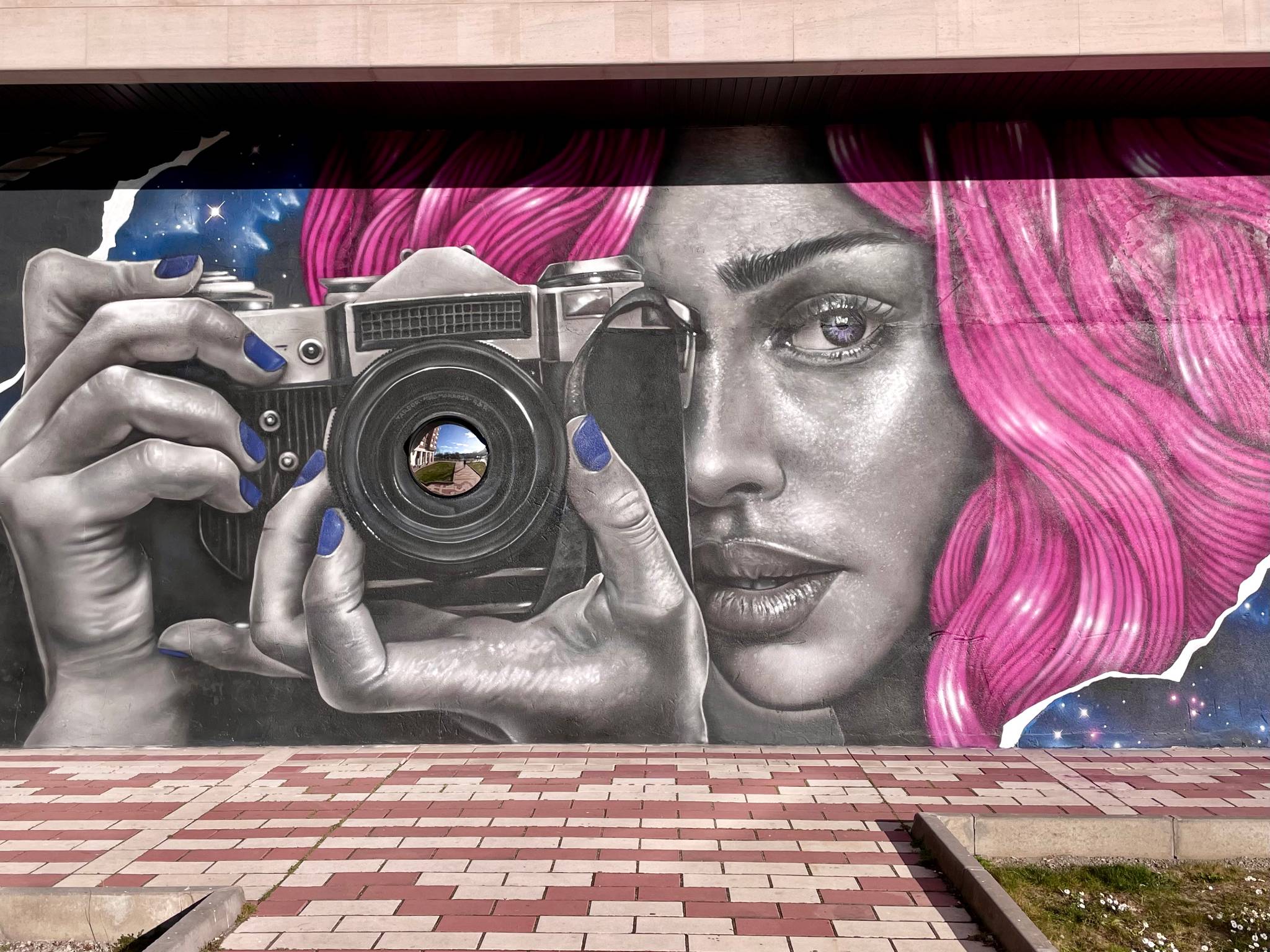The mural, displayed on the side of a building adorned with patterned pavement and clean sidewalks, is an exceptional piece of lifelike artwork. It features a young black woman in her 20s, holding a digital camera up to her face with both hands, one adjusting the dial. Her expressive face, framed by intriguingly vibrant, long pinkish-purple hair, appears to emerge from the wall, giving the impression of breaking through the cement. This three-dimensional effect adds depth and realism to the mural. Her large purple eyes and striking blue fingernails contrast sharply with the black-and-white depiction of her face and hands. Notably, the camera’s lens incorporates a real, reflective metallic surface, showing the viewer's reflection. This detail, combined with the surrounding scenes of stars and outer space in blue hues, enhances the vivid and almost surreal quality of the artwork. Patches of grass and sporadic flowers at the base of the wall complete this captivating street scene.